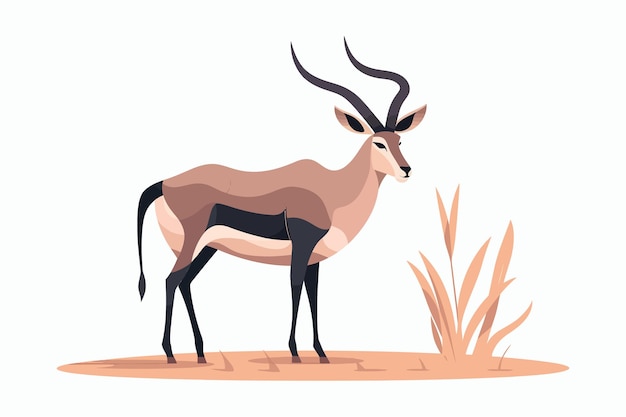An animated scene depicts an elegant deer standing on a tan-colored dirt path. The deer features a rich brown coat with a contrasting black underbelly, complemented by beige markings. The path is dotted with small plants sprouting out of the ground, adding to the natural setting. Every element in the image is upright, contributing to a serene and balanced composition. This beautifully illustrated moment appears to be taken from a book or could serve as a detailed still shot in an animated film.